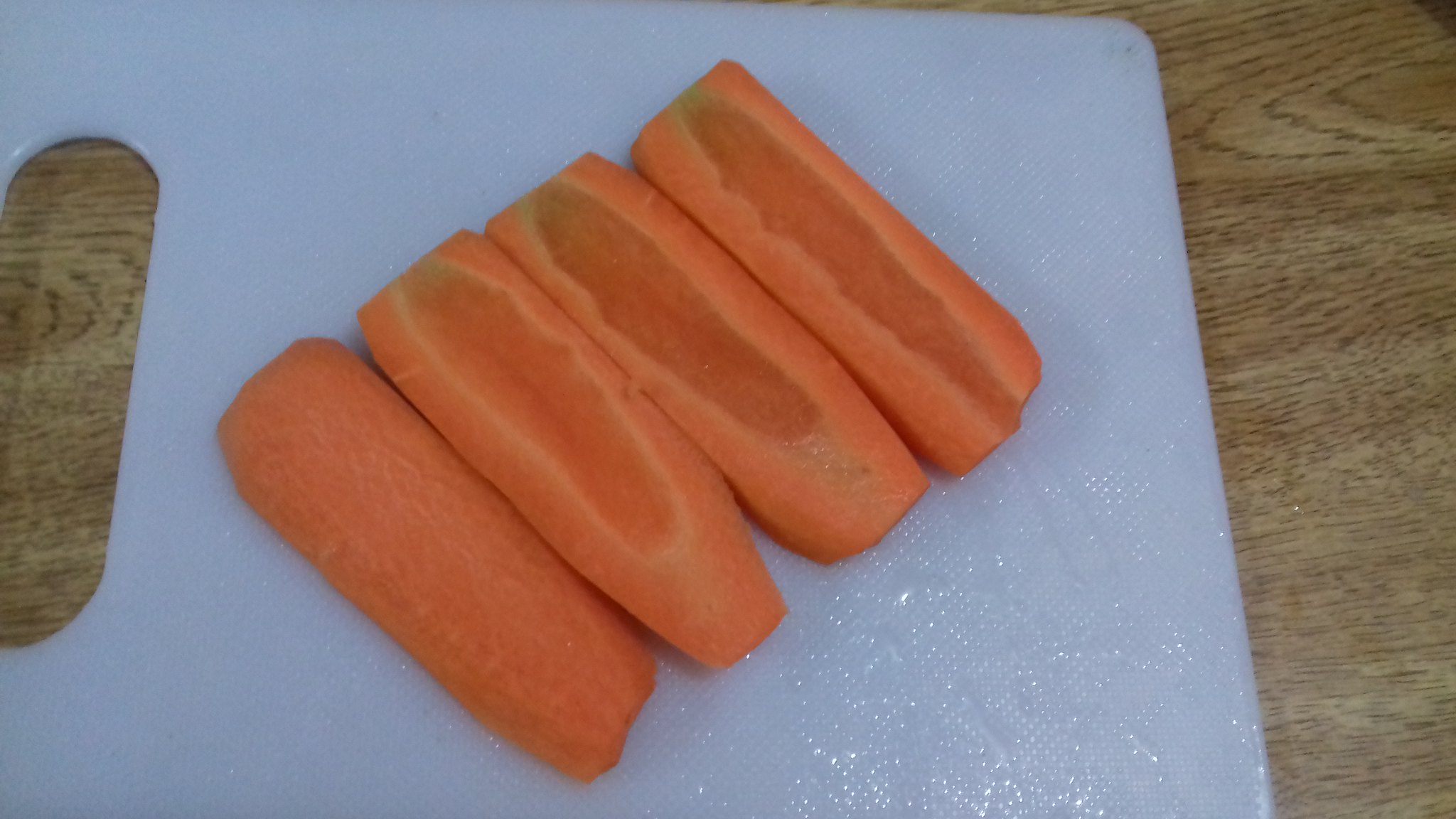The image features four slices of carrots, exhibiting a range of colors from bright orange to dark orange at the core. These evenly cut pieces likely originate from two carrots, sliced in half and arranged on a small, wet white plastic cutting board with a handle. The handle is an oblong circle through which the wooden table beneath is visible. The cutting board is situated on a light to dark brown wooden surface. The arrangement of the carrot slices extends from the bottom left to the top right, with one piece facing cut side down in the lower left corner, and the remaining three pieces positioned cut side up. The sliced carrots display slight green edges and appear to be moist, possibly indicating recent refrigeration. A reflective wet area below the cutting board suggests water or moisture present around the carrots, adding a dynamic and fresh appearance to the scene.